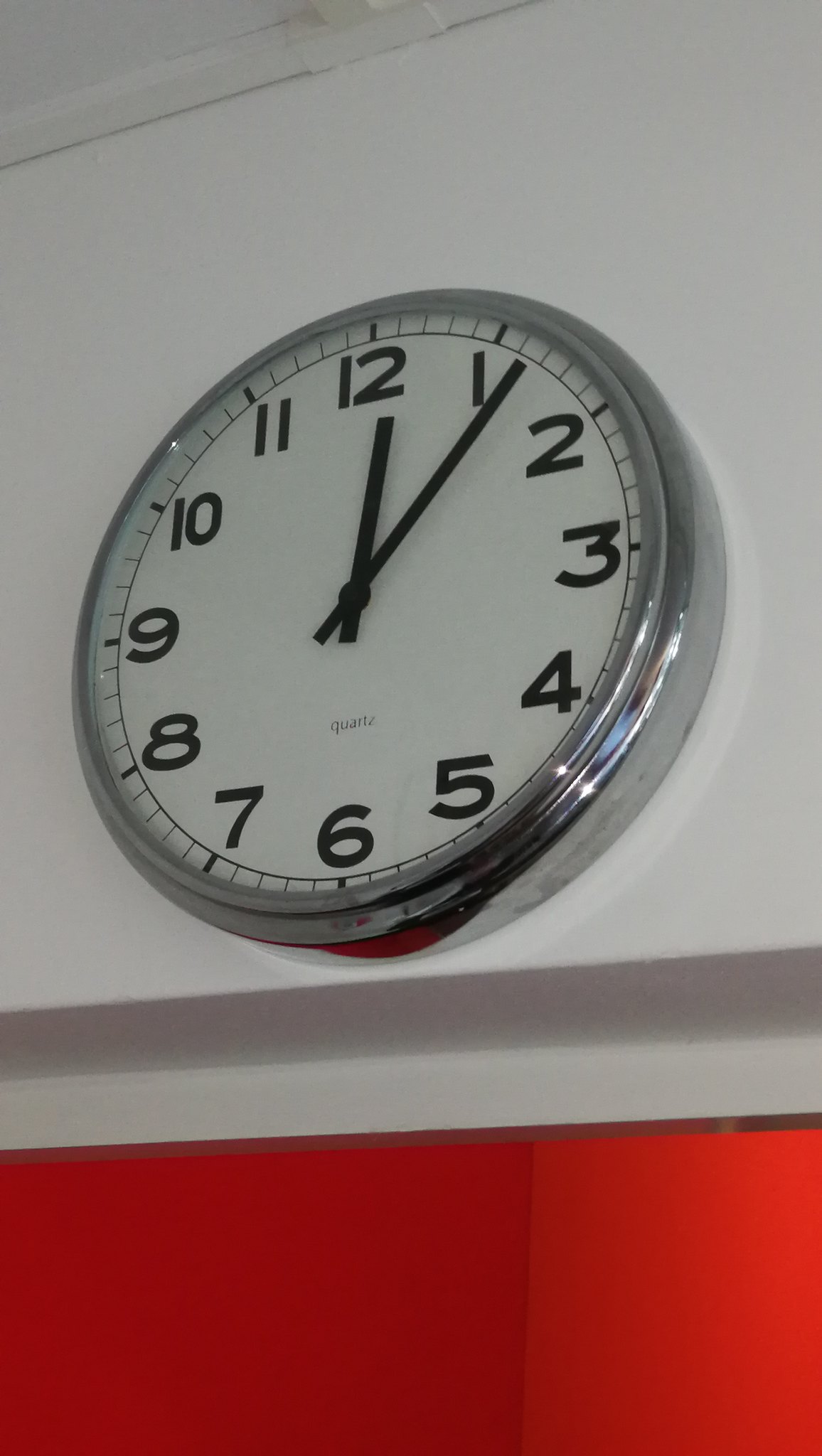This photograph showcases a silver-framed wall clock hanging on a predominantly white wall. The clock, slightly angled to face the left, features a round, smooth chrome frame with a white face, black numbers, and black hour and minute hands. It reads approximately 12:07. Positioned at the center of the image, the clock sits just below the top left corner, where a small portion of the white ceiling is visible. Below the clock, the wall is divided into a white section and a red section, separated by thin horizontal strips of gray and white molding. This red area could either be another portion of the wall or a door. The overall wall appears flat with minimal dimension, and shadows cast around the clock add subtle depth to the scene. The word "quartz" is also visible in small lettering beneath the hands of the clock.